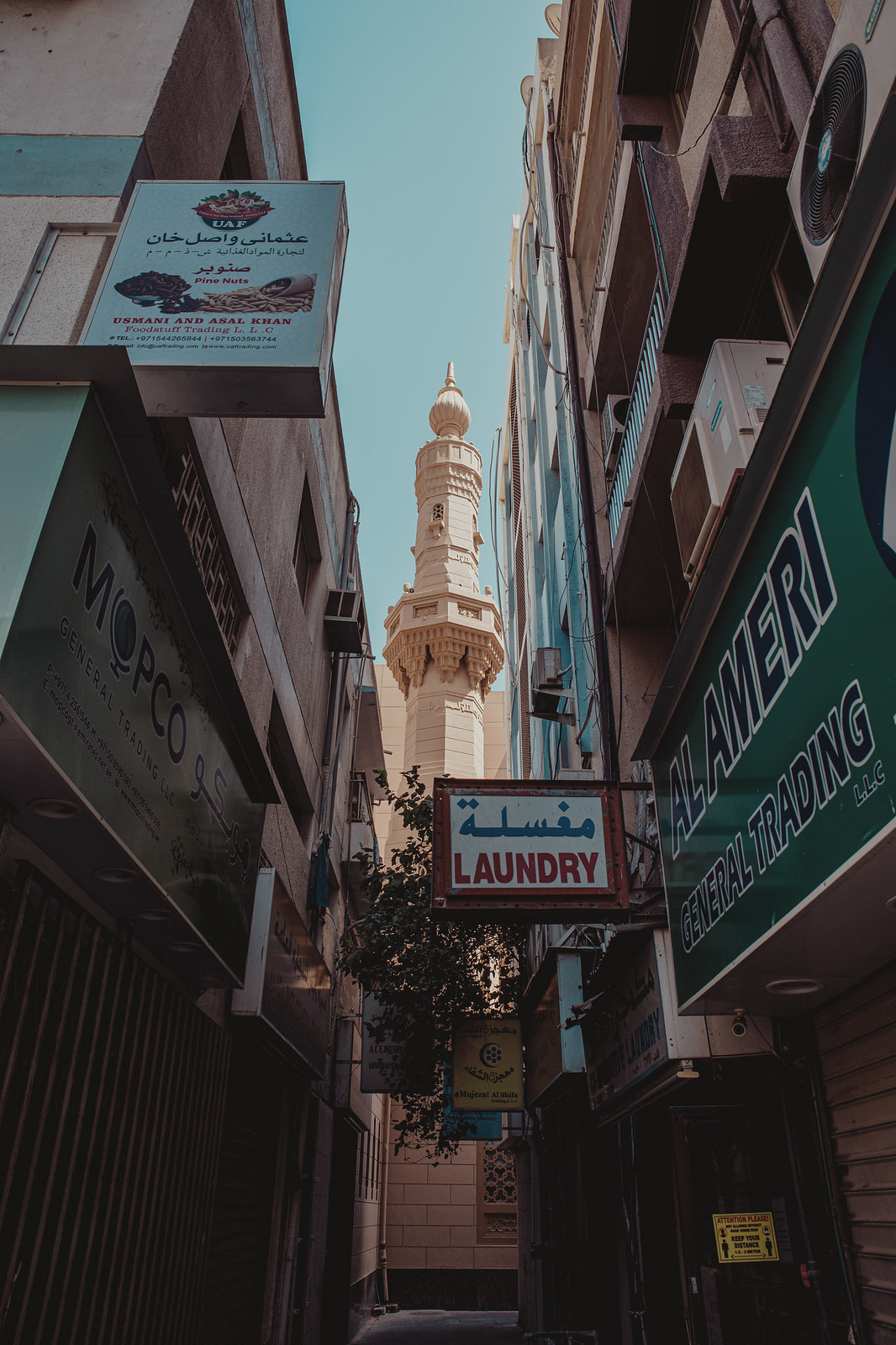This photograph features a narrow, clean alleyway in a Middle Eastern city, characterized by tall, elegant buildings on both sides. On the left, there are shorter two-story structures, including a restaurant, while the right side boasts taller, multi-story edifices. The alley is flanked by storefronts, with signs in both English and a foreign language, indicating various businesses such as a laundry store and a general trading shop. Notably, the right side of the image shows an air conditioning unit attached to one of the buildings, along with a distinctive wooden doorway. The most striking feature of the photograph is a tall, beige tower at the end of the alley, resembling a mosque minaret, with an elaborate design, a round dome, and a pointed top. The sky above is clear and blue, enhancing the vibrant but serene atmosphere of the scene.